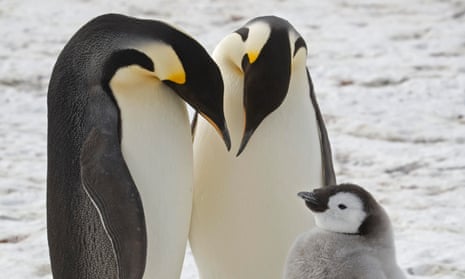In this photograph, three penguins are prominently displayed against a snowy and rugged backdrop, with indistinct hints of the ocean in the distance. The two adult penguins, positioned to the left, are characterized by their stark black and white coloring, accented with yellow patches near their cheeks. The penguin on the far left faces to the right, while the other adult, standing in the center of the image, faces the viewer directly, though both adults gaze downward at the baby penguin with evident affection. The baby penguin, situated to the right, stands out with its fuzzy gray fur and black and white head. It gazes upwards towards the adults, establishing a tender connection. The snowy ground starkly contrasts with the penguins' vivid colors, creating a striking visual of family unity in a harsh, wintry environment.